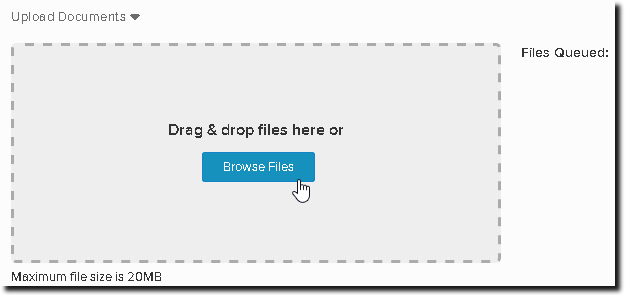The image is a screenshot of a webpage displaying a file upload interface. At the center of the image, a small hand cursor hovers over the corner of a blue rectangular button, labeled "Browse Files." Just above this button, there is an instruction reading, "Drag or drop files here." This indicates that users can either click the button to browse for files or drag and drop their files into the designated upload area. The upload area is defined by light gray, dotted lines forming a large rectangle. In the top left corner of the image, there is a link labeled "Upload Documents," accompanied by a small, downward-pointing dark arrow, suggesting a dropdown menu or additional options. In the bottom left corner, a note specifies that the maximum file size for uploads is 20 MB (megabytes). The background of the webpage is entirely white, creating a clean and simple interface focused on facilitating file uploads.